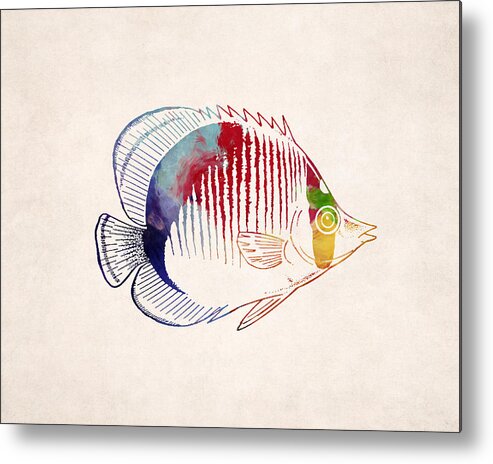This square painting features a fish at its center, set against an off-white, slightly mottled background with hints of pink, violet, and gray. The canvas is framed by a very narrow, dark-colored border that casts a shadow on the wall. The fish, oriented to the right and shaped somewhat like a spade, displays an array of vibrant colors. Its head showcases a red stripe that transitions into green near the perfectly round eye, which is outlined in white and contains a mix of green, yellow, and red. The fish's mouth is small and beak-like. Moving towards the back, red stripes begin to streak vertically before blending into blue near the tail. The fish also has distinctive, razor-sharp fins and an orange-outlined bottom fin, enhancing its abstract and vivid appearance.